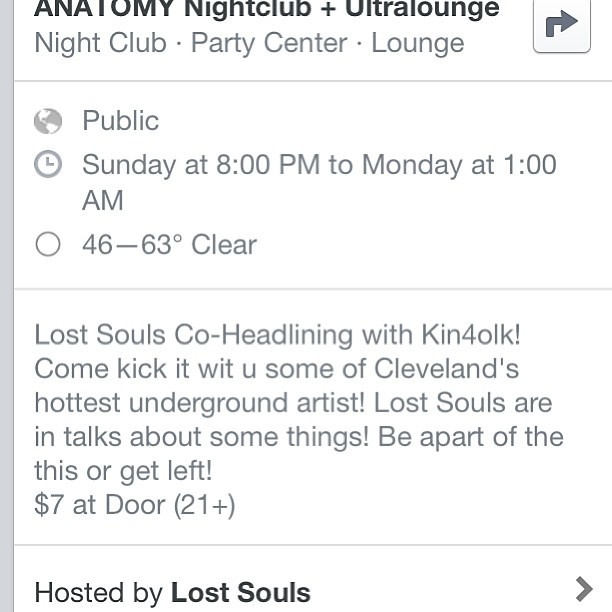**Event Invitation: "Anatomy Nightclub + Ultra Lounge" - Featuring Hottest Underground Artists**

This event screenshot showcases a social media invitation for a lively nightclub gathering. At the top of the image, bold black text announces "ANATOMY" followed by "Nightclub plus Ultra Lounge" and "Nightclub Party Center Lounge" in gray text. On the right-hand side is a button outlined with a right-pointing arrow. Below this, a light gray line separates the top section from the details below.

The event is public, indicated by a light gray Earth icon, scheduled from Sunday at 8 p.m. to Monday at 1 a.m., with a forecast of clear weather and temperatures ranging between 46-63 degrees. A paragraph detailing the event follows: "Lost Souls co-headlining with Kin for Oak! Come kick it with some of Cleveland’s hottest underground artists. Lost Souls are in talks about some things. Be a part of this or get left!" Entry is $7 at the door and restricted to those 21 and over.

The final section, separated by another gray line, notes that the event is hosted by Lost Souls, with "Lost Souls" in bold and a right arrow at the bottom right of the image. This invitation encourages participation in a vibrant night featuring significant local musical talents.